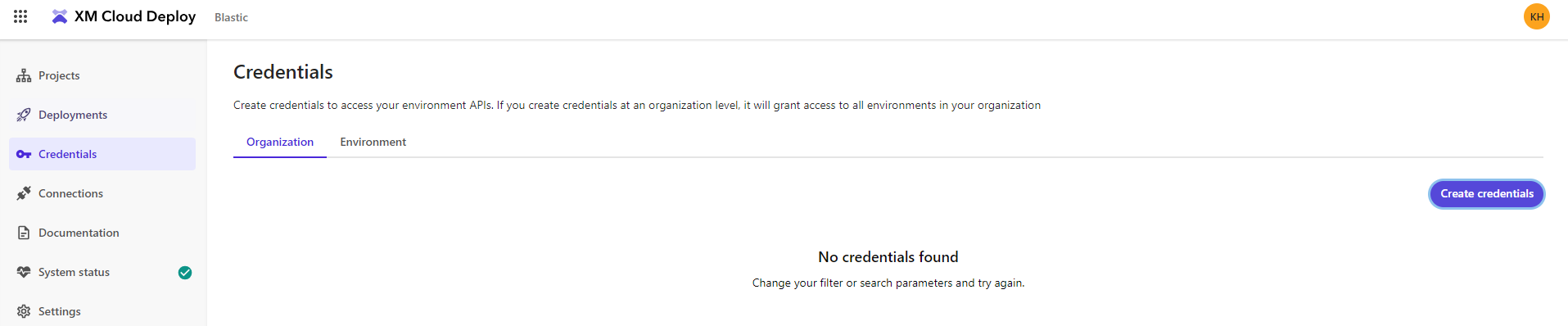This image is a detailed screenshot of a website interface. The text is very small, but in the top-left corner, it reads "XM Cloud Deploy Bait Plastic." However, it's actually "Deploy," not "Display". An orange circle containing the letters "KM" is present in the far-right corner. 

On the left side, directly under "XM Cloud Deploy," there is a vertical menu featuring a list of categories: Projects, Deployments, Credentials, Connections, Documentation, System Status, and Settings. The "Credentials" category is highlighted.

Next to the category list, a green circle with a white check mark indicates "System Status." The main panel displays the "Credentials" section, which provides a message: "Create credentials to access your environment APIs. If you create credentials at an organization level, it will grant access to all environments in your organization." There are two tabs available: "Organization" and "Environment," with "Organization" currently highlighted. The message "No Credentials Found. Change your filter or search parameters and try again." is displayed in this section.

On the right-hand side, there is a bright "Create Credentials" button. Additionally, in the top-left corner next to "XM Cloud Deploy," there's an icon consisting of three rows of three dots forming a square.